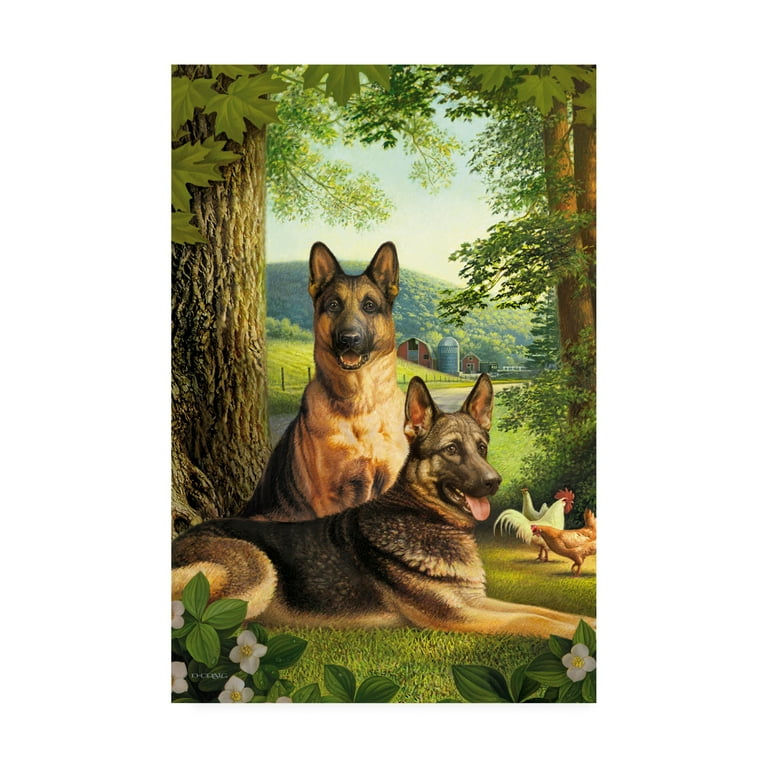This beautifully detailed painting captures a serene nature scene. In the foreground, two German Shepherd dogs are prominently positioned. The dog in front is sitting and facing slightly to the right, with its head turned forward and its tongue playfully hanging out. The second German Shepherd stands alertly behind the first, its front legs upright and its mouth open. Both dogs have erect ears and exhibit a striking golden brown coat with darker brown accents along their backs.

Adjacent to the dogs on the left-hand side, a tree rises with a sturdy trunk and an abundant canopy of what appear to be maple leaves. On the right-hand side, set slightly further back, stands another tree with a distinct type of foliage, beneath which several chickens are perched.

The foreground is adorned with patches of white flowers interspersed with lush green grass, adding a touch of elegance to the scene. In the background, behind the dogs, stretches a tranquil pasture enclosed by a rustic fence. A vibrant red barn adds a splash of color, while a gently rolling hill covered in a thick forest of trees extends towards the horizon. The overall setting is bathed in the warm glow of a sunny sky, suggesting a peaceful, idyllic afternoon.